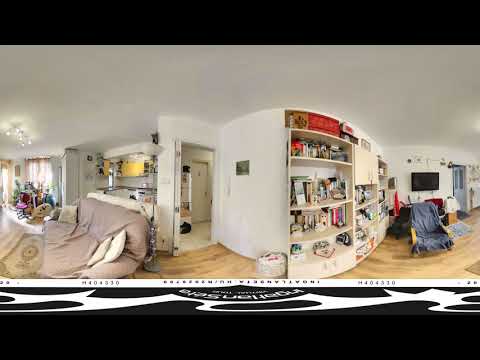This is a small, horizontal, rectangular photograph of an indoor setting taken with an unusual lens, causing noticeable distortion in the shapes. The image is bordered by thick black bars at the top and bottom, with the bottom bar containing unreadable upside-down writing. The scene appears to capture the inside of a house or possibly an apartment with a cluttered arrangement of various household items. On the left side, there is a kitchen countertop that possibly divides the room, with either windows or a door allowing a lot of light to pour in. Adjacent is a couch accompanied by a rug on what seems to be a hardwood floor, and a nearby lighting fixture beside a window with drapes.

Moving toward the center, the image seems to feature a foyer area leading to a main door, flanked by storage shelves in a lighter cream or beige color against white walls and ceiling. On the right side, there are multiple objects including a wall-mounted TV, a chair with a blue cover, a photograph, and a vehicle-like shape suggesting a garage-like space or another open area. The entire setting exhibits a mishmash of items like carpets, bookstands, and an assortment of colors including shades of black, white, brown, blue, purple, red, yellow, orange, and gray. Amid the distortion and clutter, the image seemingly portrays an indoor scene during daylight hours.